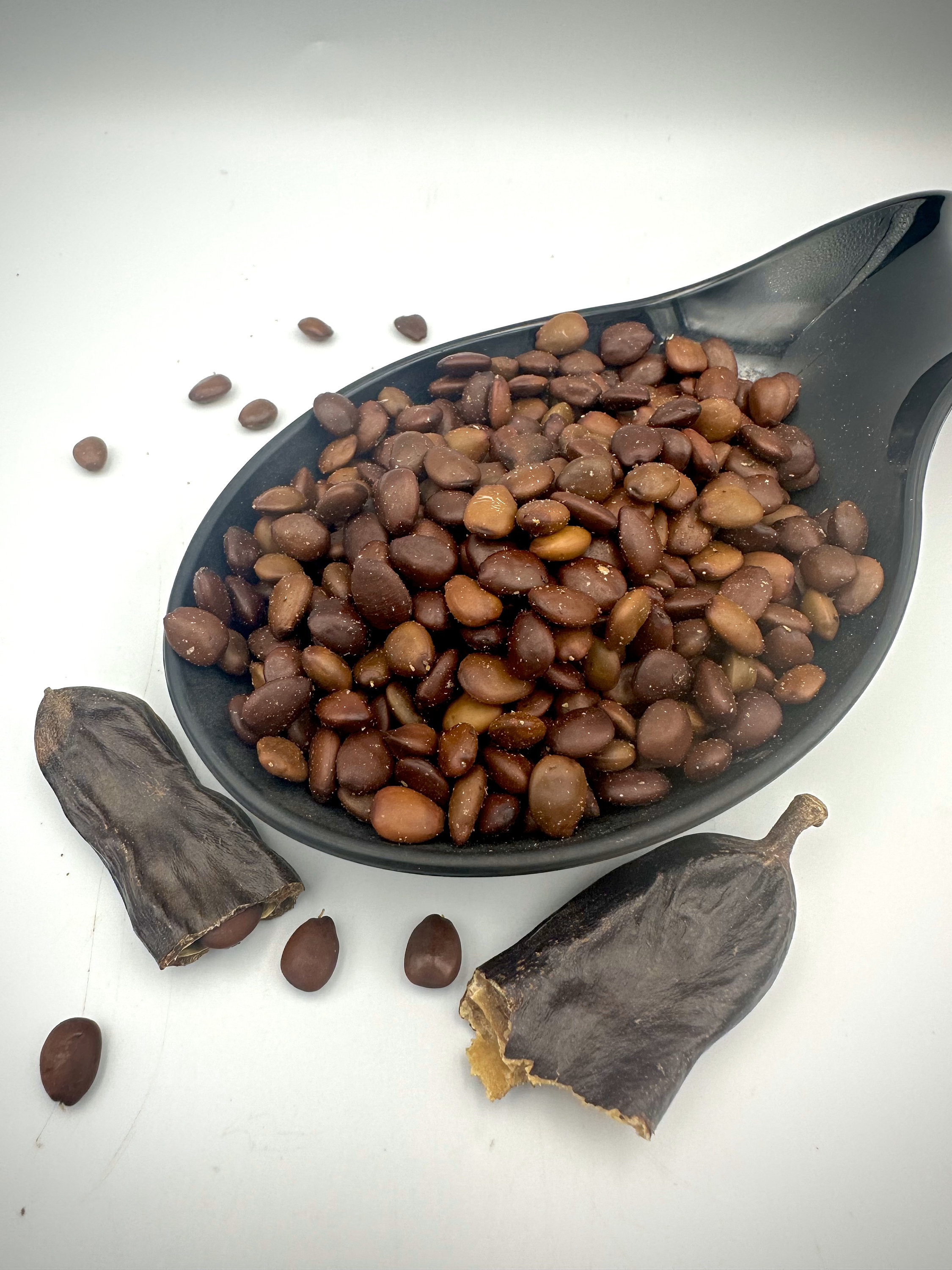In the photo, we see a large, spoon-shaped dish with a handle that resembles a ladle or cooking utensil placed on a solid white table. The dish, which is black, features a wide, circular top that tapers to a narrow end. Inside the dish, there's an abundance of small, nut-like chocolates, varying in shades of brown and featuring small white spots, indicating they might have been processed or slightly nicked. Surrounding the dish are a few scattered chocolates, adding to the sense of a generous amount. In front of the dish, there are two large, flat, light-brown pods, one of which is split open, revealing some of the chocolates inside, while the other appears empty with a visible stem. The background is white and appears slightly grayish at the top and bottom, emphasizing the focus on the dish and its contents.